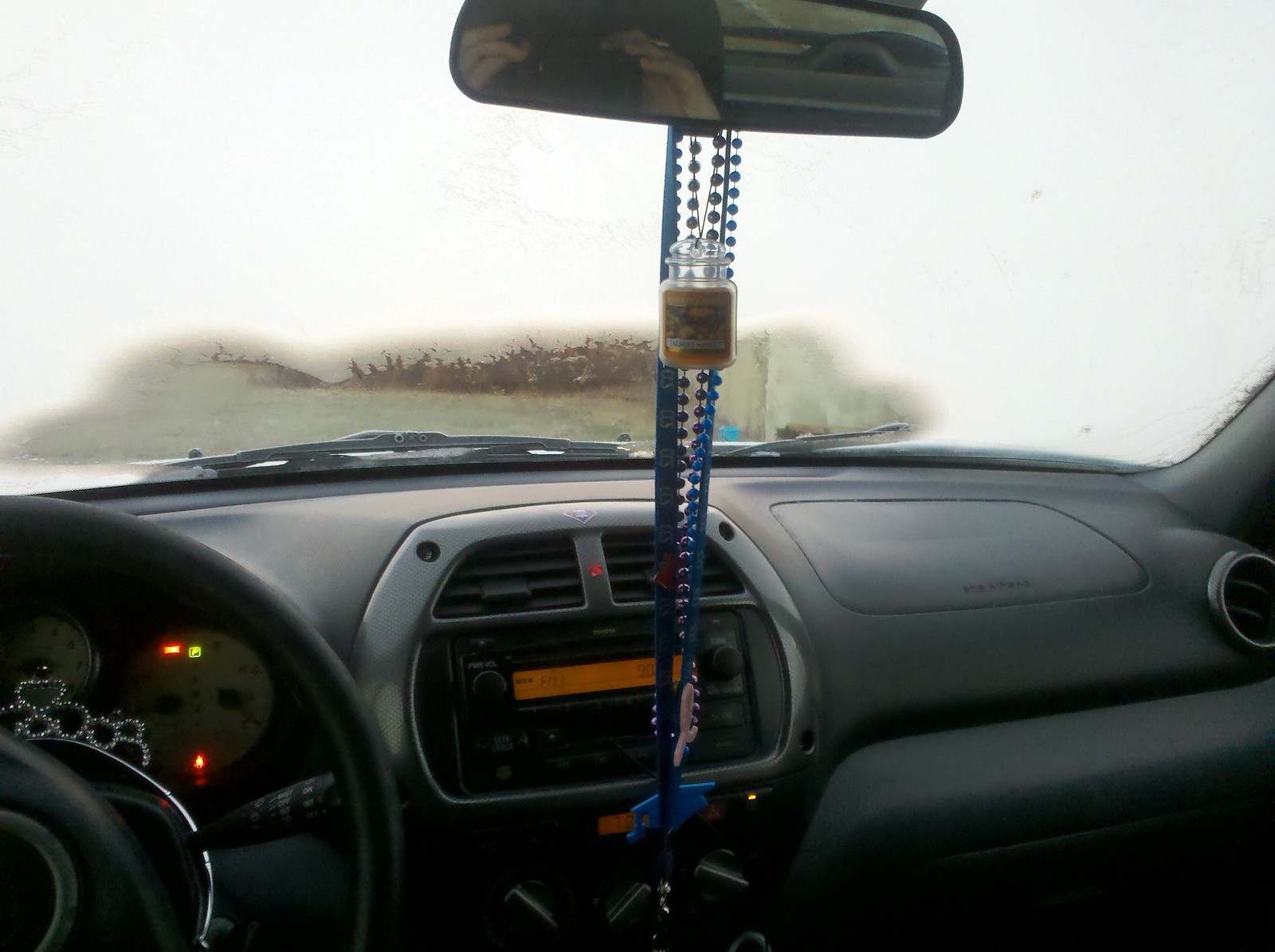The photograph captures an interior view from the driver's seat of an older model car. The central focus is on the steering wheel, dashboard, and fogged-up windshield, which has a small defrosted area near the windshield wipers. The car's dashboard features a basic, curved design with a stereo sporting an older style orange display, flanked by two air vents at the top. Various dashboard lights are illuminated, including a check engine alert, seatbelt warning, and a green "park" indicator, confirming the car is parked.

In the upper part of the frame, the rearview mirror is adorned with beaded necklaces, a lanyard, and a Yankee Candle air freshener. The camera's reflection, along with the photographer's hands, is visible in the mirror. Part of the gray dashboard also incorporates white gauges, and the left side of the steering wheel appears cut off by the photo’s edge. Over the top of the wheel drapes a silver tiara resembling a New Year’s Eve crown.

The icy windshield displays a textured pattern indicating frost and snow, most noticeably concentrated on the upper right side, with the defrosted area centralized at the bottom middle above the wipers. Due to the heavy frost, visibility through the window is almost nonexistent, framing an impression of a cold, wintry day outside.